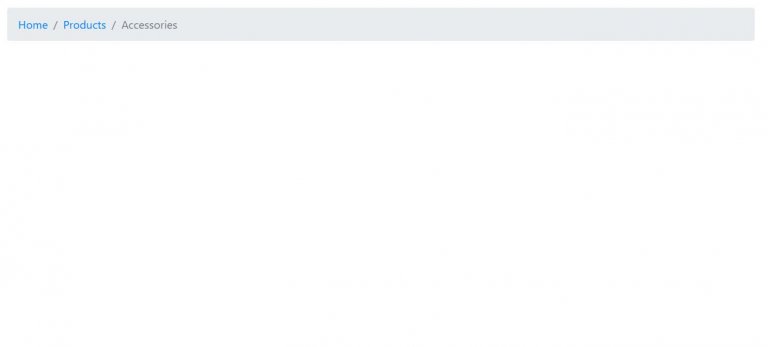Website Screenshot Description:

The image showcases an unfinished or partially loaded website. The overall color scheme appears predominantly grey, with a starkly white background. At the top of the page, there's a navigation bar featuring the categories: "Home," "Products," and "Accessories," each separated by a slash. The navigation text is grey, except for "Home," which is highlighted in blue, indicating it is the currently selected or hovered-over option.

The word "Accessories" is distinctly formatted in all uppercase letters: "ACCESSORIES." Despite the visible elements, the rest of the page appears empty or not fully loaded, offering no additional content or visual details to comment on. The simplicity and lack of content suggest that the website might be in the process of loading or still under development.